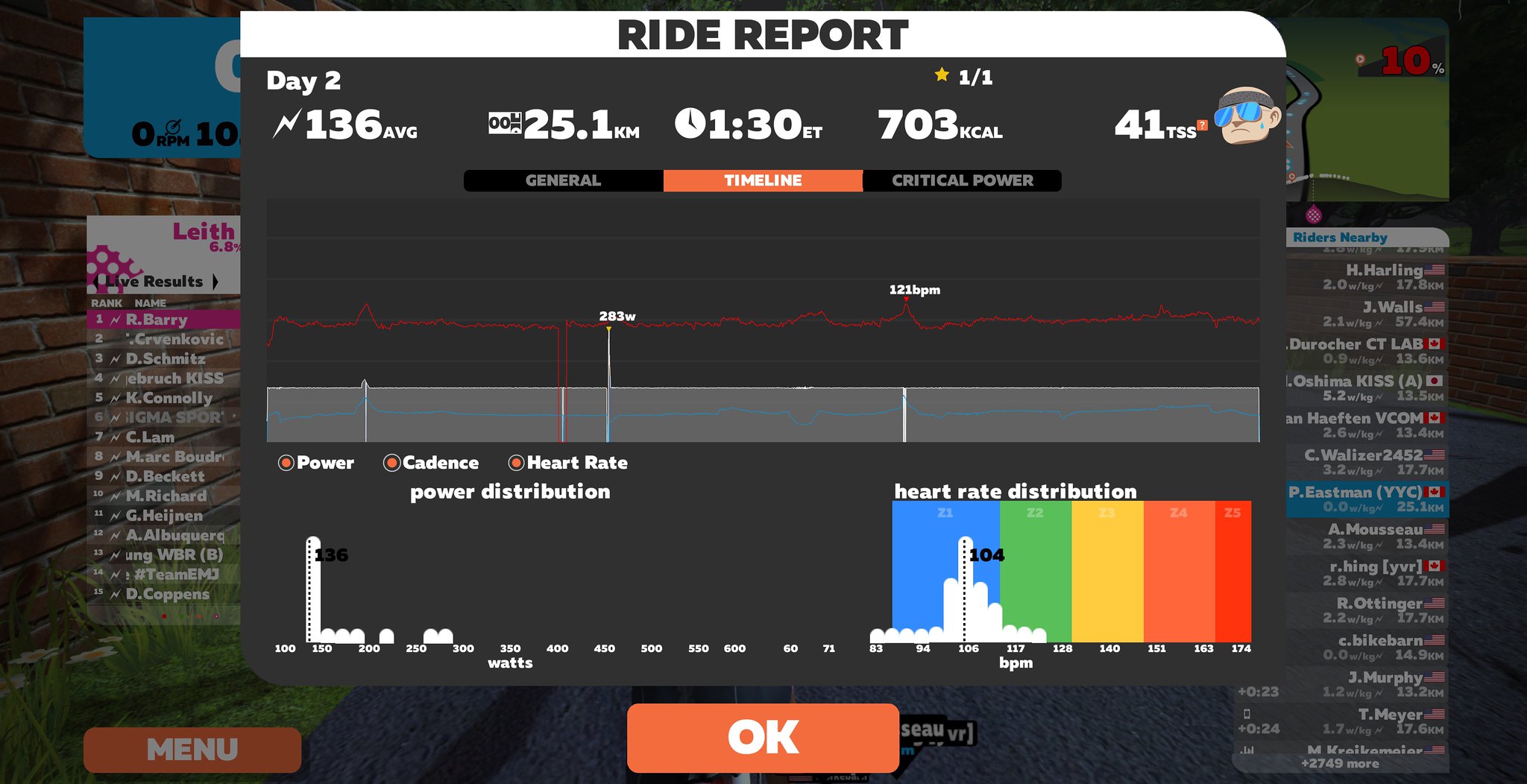The image is a detailed screen capture from a fitness app focused on cycling, showcasing a ride report. At the top center, bold black text reads "Ride Report," with "Day 2" highlighted beneath it in white. The report presents various statistics: an average speed of 136, a distance of 25.1 kilometers, and a time of 1:30 ET. It also notes that the rider burned 703 kcal and achieved a Training Stress Score (TSS) of 41. In the upper-right corner, it indicates "1 of 1" and displays a small cartoon of a white male with a black headband and blue sunglasses.

Central to the image, headings labeled "General," "Timeline," and "Critical Power" categorize the data. Below these headings is a prominent line graph, mostly flat, with key data points marked as 121 BPM (beats per minute) and 283 W (watts). Further down, two bar graphs measure power distribution, heart rate distribution, and potentially cadence.

Along the bottom of the Ride Report, the screen offers more detailed metrics under the labels "Power," "Cadence," and "Heart Rate." Accompanying these is a heart rate distribution histogram, detailing different heart rate zones achieved during the ride. Additional elements include an OK button to dismiss the report and background information on nearby riders and the individual’s travel routes. Together, these components provide a comprehensive summary of the cyclist's performance.